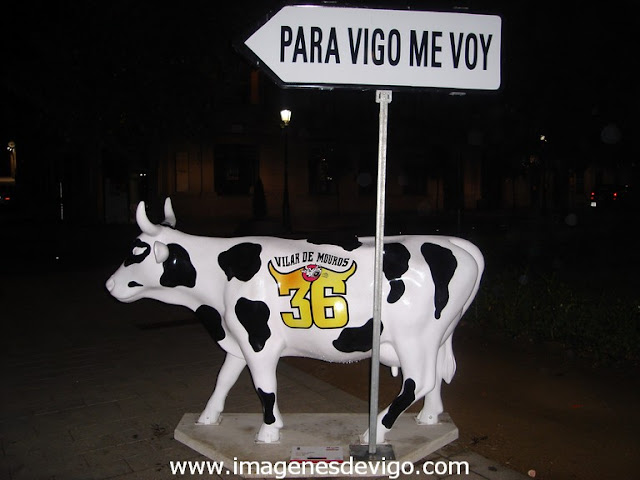This nighttime photograph captures a striking black and white cow statue standing on a dirty white, hexagonal platform. The cow's body features the text "Villa de Mars" prominently in black, with the number 36 positioned below. The numbers 3 and 6 are flanked by two small horns each, and in the center, a red logo depicts a cow. In front of the cow, on the platform, a tall white post bears a white arrow-shaped sign with black text that reads "Para Vigo Me Voy." The sign is affixed to a silver metal post anchored into a gray plaque at the base. The background is quite dark, with only dim lighting hinting at a nearby building and the faint red glow of automotive taillights in the distance. The cow points its face towards the left, with its body extending to the right, showcasing the classic black spots on its white coat. At the bottom of the platform is the text "www.imagenestvigo.com," completing the setting in what appears to be an outdoor street scene.